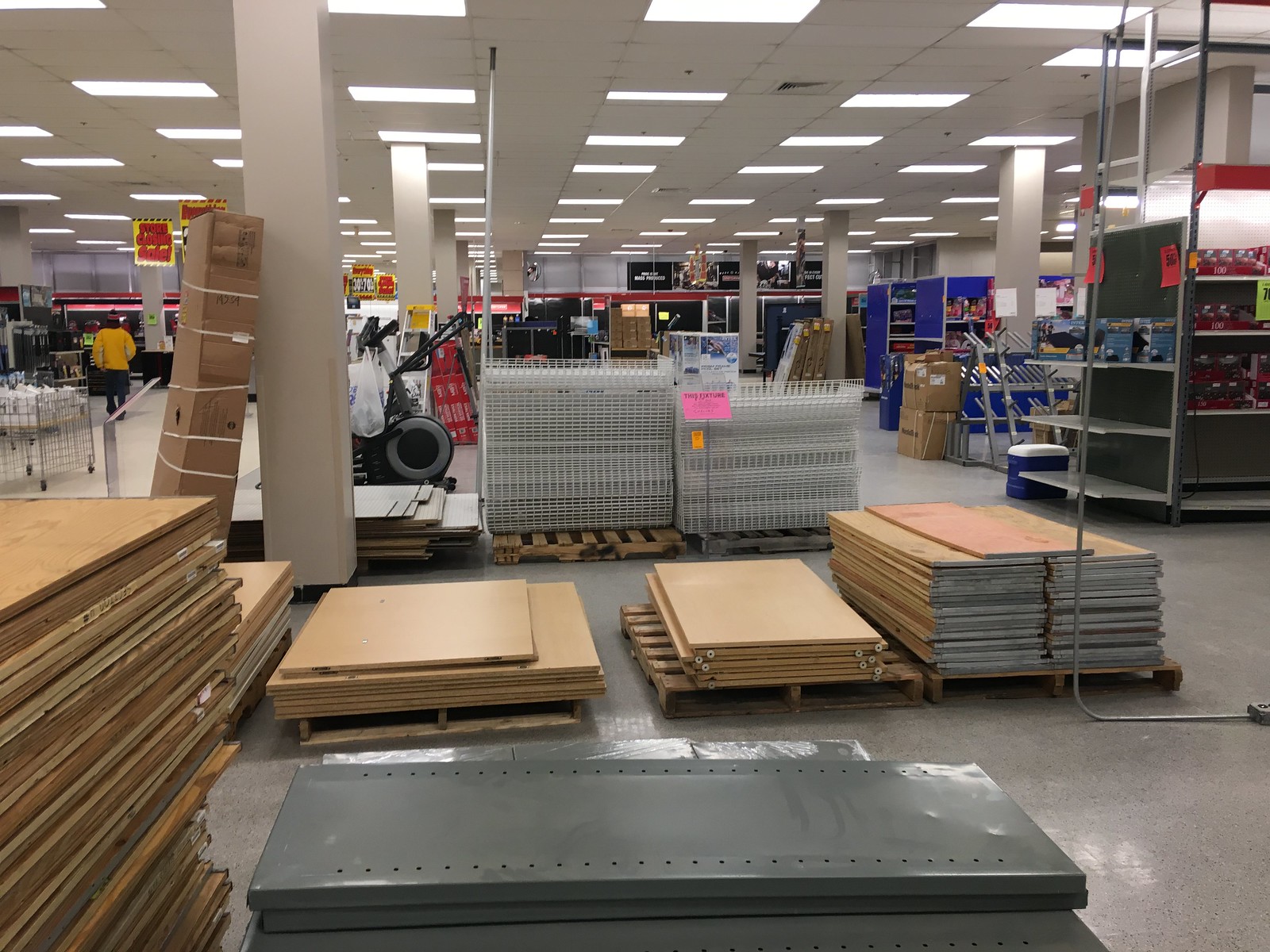The photograph showcases a store in the midst of a going-out-of-business sale. The scene is filled with partially stocked shelves, sparsely populated with remaining products. Colorful discount signs are visible throughout, displaying large percentage reductions of 50% and 70%. In the foreground, heaps of store fixtures are scattered, including detached shelving units and side pieces. Several pallets laden with shelving materials are stacked alongside more pallets bearing white metal grid fixtures. In the distant background, a series of "Store Closing Sale" signs hang from the ceiling, particularly noticeable in the top left corner, emphasizing the store's final days of operation.